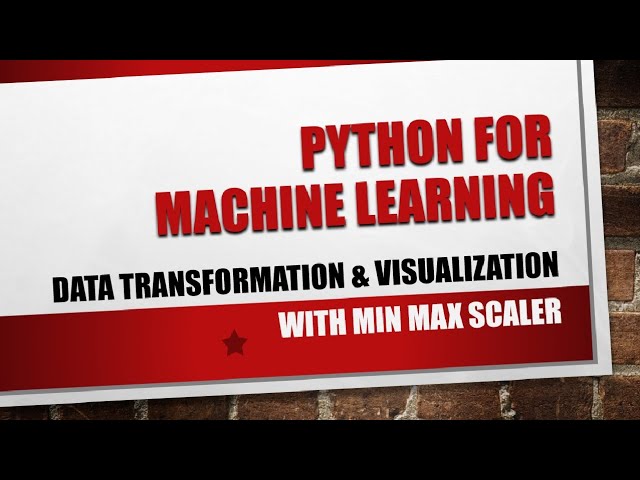The image depicts an advertisement banner positioned against a brown brick wall with visible gray cement marks. The banner predominantly features red and white colors, with a thin gray border on the sides. It includes three main sections of text, all written in all caps. The top section of the banner, which is red, prominently displays "PYTHON FOR MACHINE LEARNING" in large red letters. Below this, there is a central white section with the text "DATA TRANSFORMATION AND VISUALIZATION" written in black. The bottom section is also red, featuring the text "WITH MIN MAX SCALER" in white. Additionally, to the left of the final portion of text, there is a small, darker-colored star. The image itself has a black border framing the content.